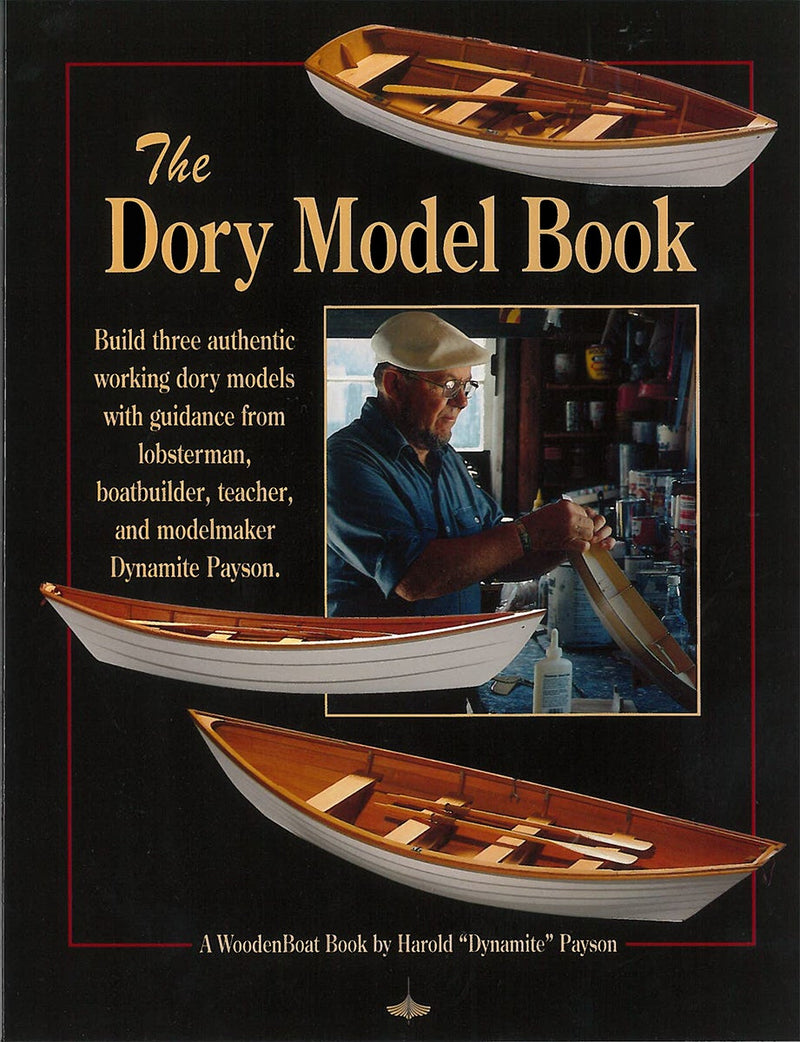The cover art of the book, titled "The Dory Model Book," predominantly features a black background with detailed illustrations and text. Central to the cover are images of three distinct dory boats, each designed as authentic working models with warm wooden interiors and two oars inside each, highlighting their careful craftsmanship.

At the top of the cover, there is a depiction of a model boat, revealing its interior with two oars and three seating areas. Below this, the subtitle reads: "Build three authentic working dory models with guidance from lobsterman, boat builder, teacher, and model maker, Dynamite Payson." This is followed by another image of a thinner model boat with white paneling and a darker, light wood interior.

Centrally, there is an illustration of Dynamite Payson himself, depicted in his woodworking shop. He is shown wearing a white cap, glasses, and a blue shirt, diligently working on a model boat which appears to be in the process of being glued together. His workshop, filled with various woodworking tools, sets the scene of meticulous model making.

At the bottom left, text reads: "A Wooden Boat Book by Harold 'Dynamite' Payson." The cover combines the sophistication of model boat crafting with Payson's expert guidance, providing a comprehensive and inviting visual preview of the book's content.